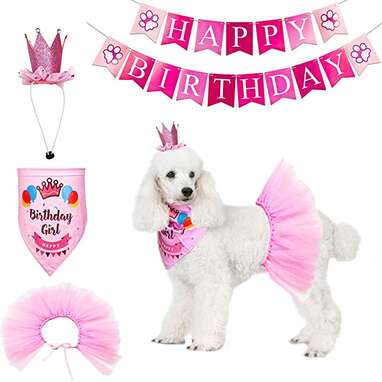The image showcases a white poodle celebrating its birthday, adorned in festive attire. The poodle, facing the camera with a cute pink crown on its head, wears a pink tutu and a pink bandana that reads "Birthday Girl," which features crown and balloon graphics in red, blue, and yellow. Its black eyes and nose stand out against its fluffy white fur. Above the poodle, two rows of bunting form a "Happy Birthday" banner, with pink paw print flags at each end and alternating shades of pink for each letter. To the left of the poodle, smaller images display close-ups of the birthday crown, bandana, and tutu, highlighting the intricate details of each accessory.